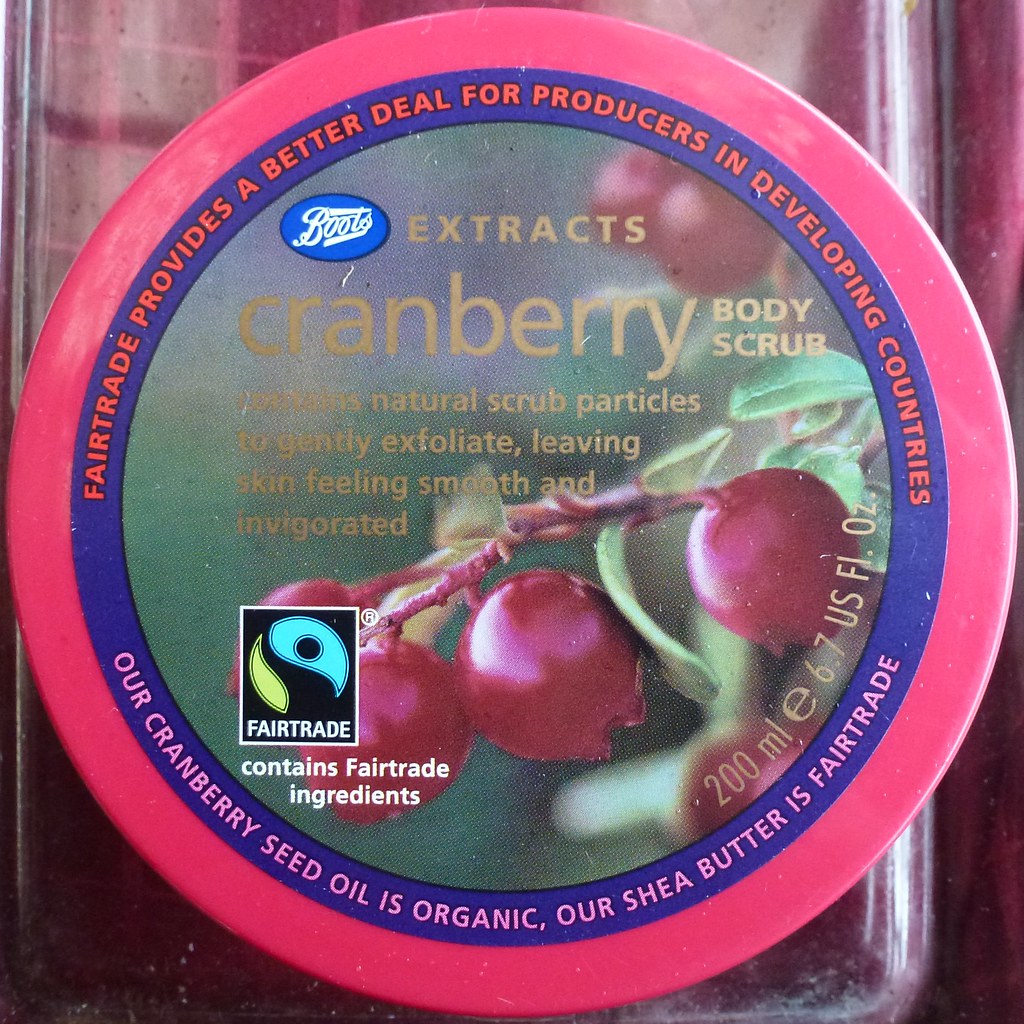The image is a top view close-up of a circular body scrub container. The outer rim of the container is pink with a blue inner ring. On the blue ring, it reads "Fairtrade provides a better deal for producers in developing countries" at the top and "Our cranberry seed oil is organic. Our shea butter is Fairtrade." at the bottom. In the center, there is a branch of red cranberries with green leaves on the right side. Above the cranberries, the brand name "Boots" is printed in white on a blue oval shape, with "Extracts" in yellow to the right. Below this, it says "Cranberry body scrub" and "Contains natural scrub particles to gently exfoliate."